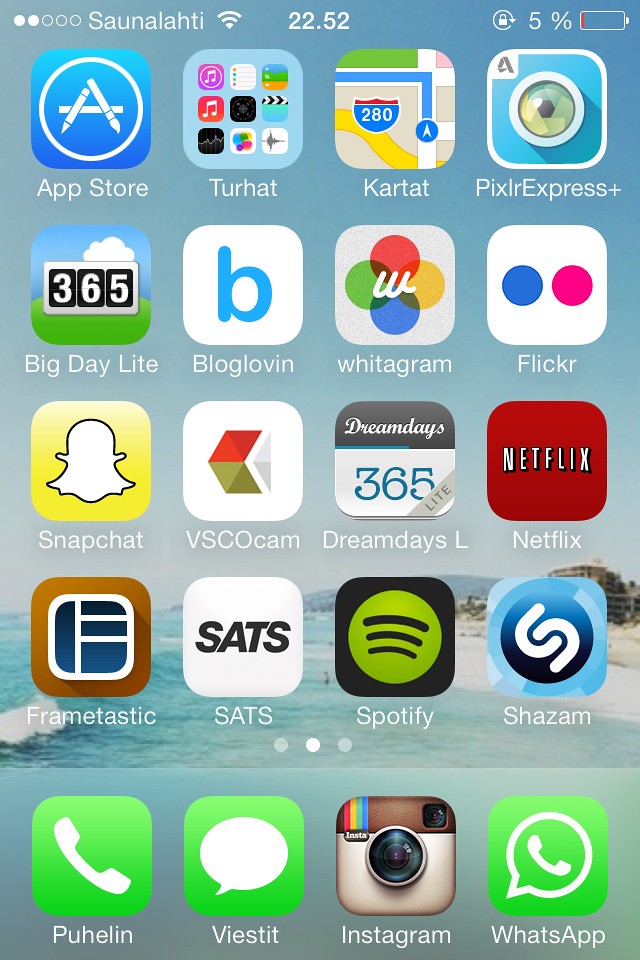The image showcases the home screen of what appears to be a Galaxy tablet, arranged with a grid of apps organized in a five-by-four layout. The apps visible include the App Store, Terhat (featuring numerous other apps), Cartat (likely a street navigation app), Pixel Express Plus, Big Daylight, Blog Lovin', Whitagram, Flickr, Snapchat, VSCO Cam, Dream Days L, Netflix, Framtastic, Stats, Spotify, Shazam, Fulin, Instagram, and WhatsApp. The background wallpaper features a serene beach scene, capturing the daylight ambiance with gentle waves rolling onto the shore.